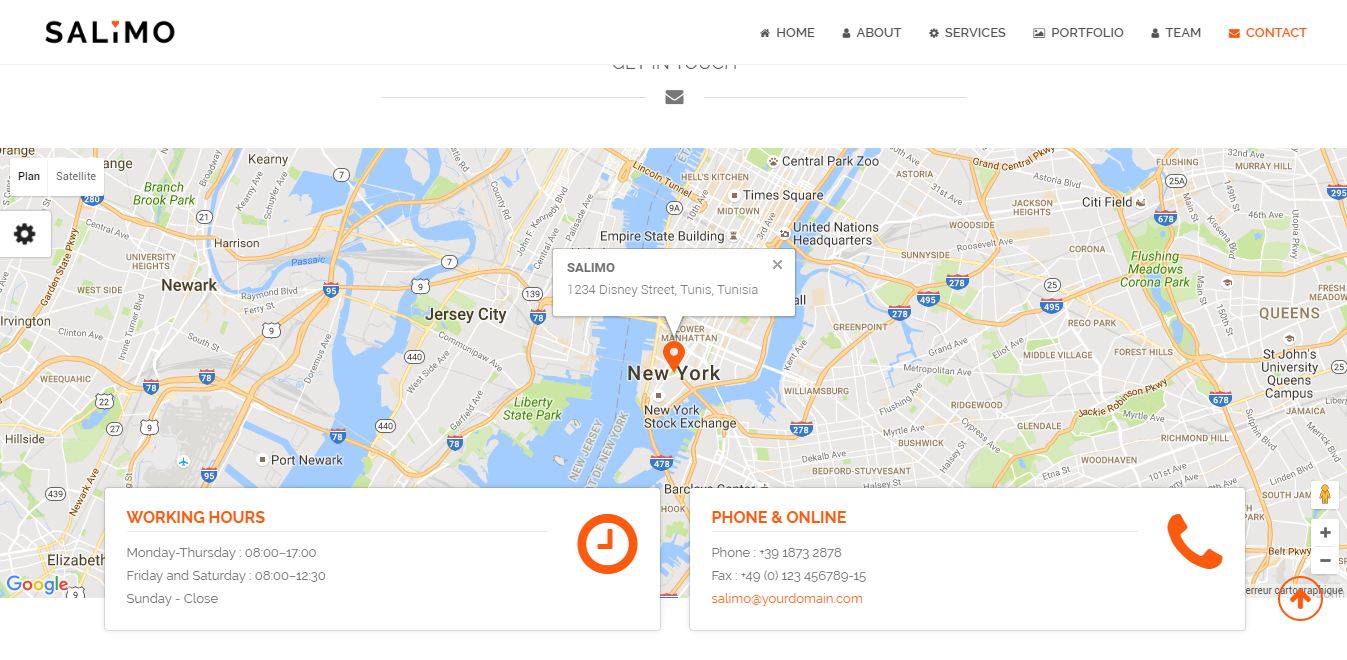The image depicts a Google search result for "Salimo," a business characterized by a lowercase 'i' with a heart for the dot in its name. This business appears to be located in Tunisia and serves the New York City area, as indicated by the map view showing parts of New Jersey, Newark, Jersey City, New York City, and Queens, including major interstates. The top navigation bar of the page includes tabs for "Home," "About," "Services," "Portals," "Team," and "Contact," suggesting a professional service business.

Salimo's working hours are detailed in a 24-hour format: Monday through Thursday from 8:00 a.m. to 5:00 p.m., Friday and Saturday from 8:00 a.m. to 12:30 p.m., and they are closed on Sunday. The contact information section prominently features an orange phone icon, listing the business's phone number, website, and fax number, while the hours section displays an orange clock icon. The map notably highlights nearby regions, emphasizing Salimo's broad service area encompassing prominent neighboring locations.